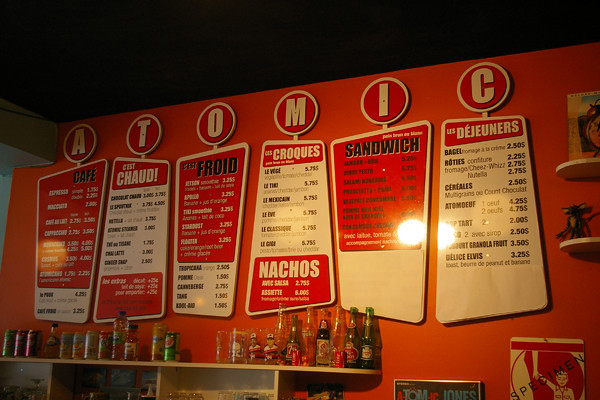The image captures the interior of a restaurant, showcasing a striking bright red wall and a black ceiling. Dominating the wall is a series of uniquely shaped signs, each featuring a combination of circular and trapezoidal elements. The circles collectively spell out "ATOMIC," with each letter serving as a header for different sections of the menu. Specifically, "A" details the café menu, "T" highlights travel-related offerings, "O" presents Freud's selections, "M" lists croquis and nachos, "I" features sandwich options, and "C" offers the Degenerous menu. The signs are distinctively designed with either a red or white background and contrasting white or black text.

Below these signs, a shelf holds various sauce bottles, glasses, and cans, adding a touch of practicality and decoration to the space. To the right of the signs, another shelf is visible, adorned with a figurine and a painting, further enriching the eclectic and vibrant ambiance of the restaurant.